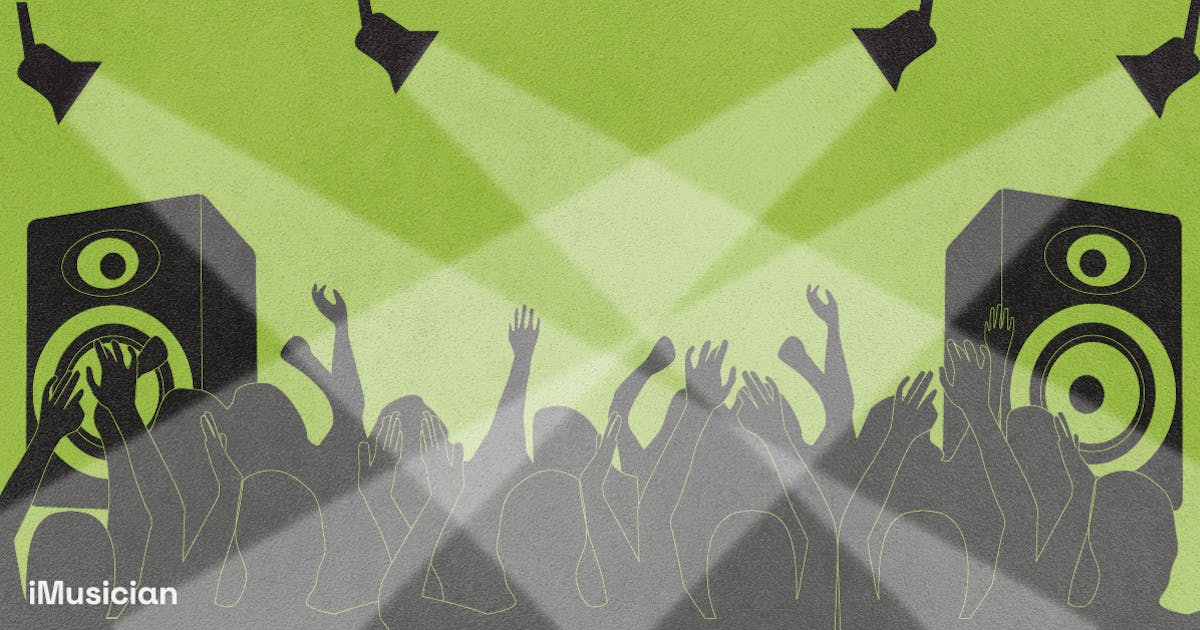This graphic illustration serves as a lively promotional ad, possibly for a music-related venue, service, or software called "iMusician." The image, rendered in a minimalist and cartoonish style, features a forest green background. At the center of the illustration, an enthusiastic crowd of silhouetted people with hands raised suggests the atmosphere of a concert or rave. Flanking the crowd, two large black speakers stand on either end, while four spotlights positioned above cast beams of light downwards, enhancing the concert-like feel. The lower left corner prominently displays the brand name "iMusician," indicating its promotional intent. The overall composition and animated design make it suitable for website use or other digital advertising mediums.